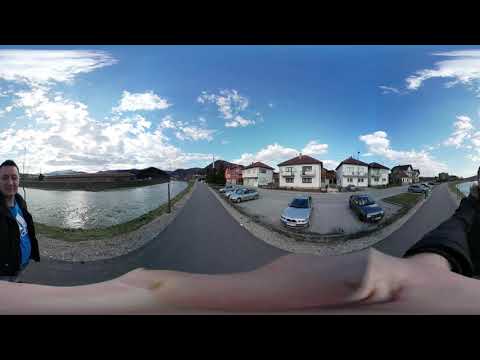This panoramic photo showcases a bright blue sky with a few clouds, capturing a vivid scene of contrasting elements. To the left, a man with dark hair, wearing a blue Adidas t-shirt under a black jacket, stands by the edge of a body of water. The water stretches partway across the scene before transitioning into a roadway that runs through the center of the image. On the right side of the road, a parking lot houses six cars, backed by white buildings with brown roofs, suggesting residential houses. A lingering detail in the bottom left shows the man's side profile, cut off at the waist, while his warped, outstretched hand and a sleeve-clad arm reappear on the right, adding a curious distortion to the otherwise serene landscape. Black framing borders the top and bottom of the photo, hinting that it was taken with a 360-degree camera, adding depth to the bright and detailed composition.